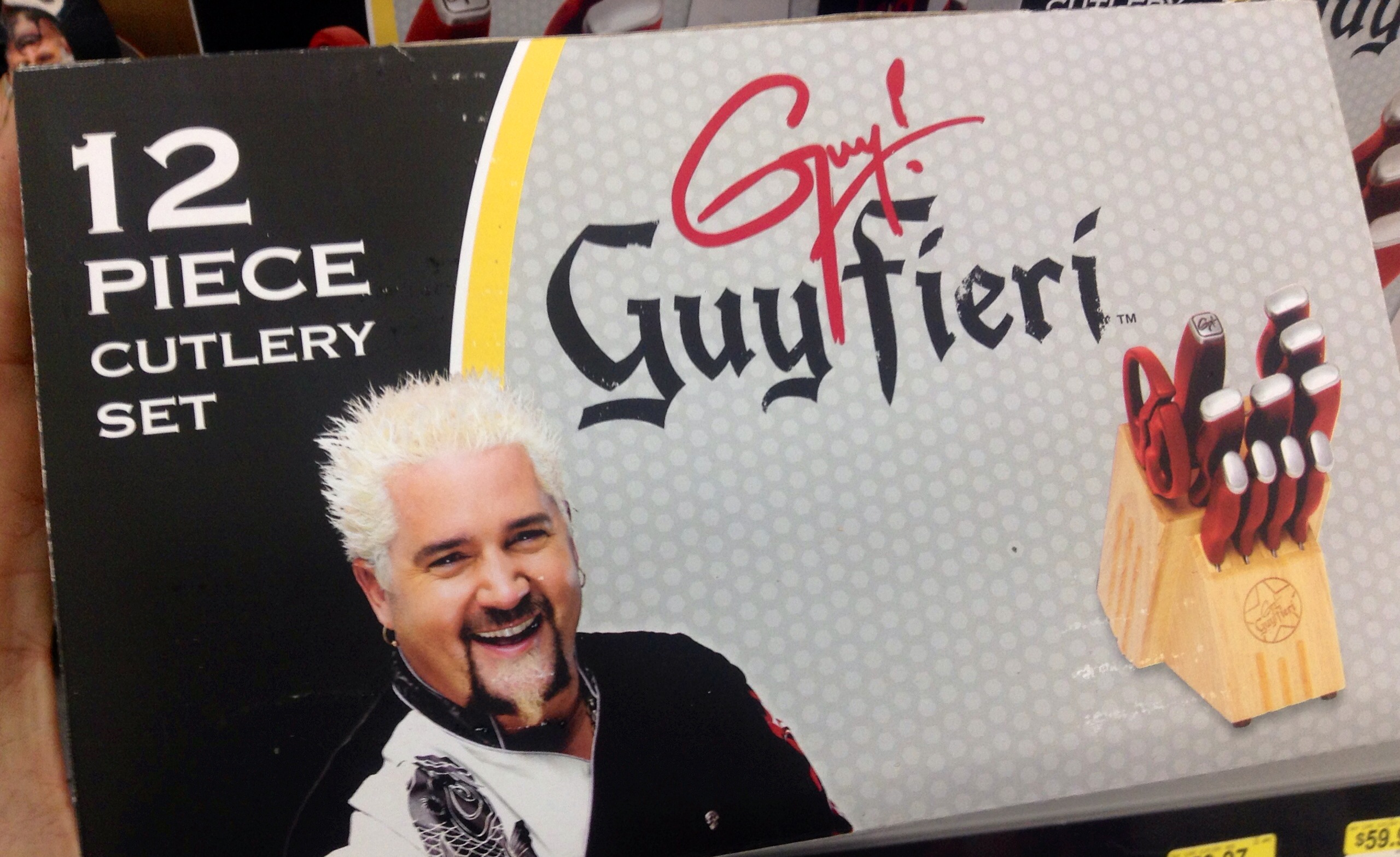This image is an advertisement poster board for a Guy Fieri sponsored 12-piece cutlery set. The background features a distinctive design: the left one-third is black with a yellow stripe running down, while the right two-thirds display a gray honeycomb pattern. Prominently displayed on the top left section in bold white text are four lines stating "12-piece cutlery set." Just below the text, there's a picture of Guy Fieri, captured from mid-chest up, with his signature spiked bleach-blond hair, black and white goatee, and a hint of a white beard. He is smiling broadly, dressed in a black and white top adorned with a koi fish design and sporting an earring. His name appears twice on the poster: in larger red letters "Guy!" followed by "Guy Fieri" in black. On the lower right side of the poster, an image of the cutlery set is displayed, featuring a set of dark-handled knives neatly arranged in a wooden block, complete with a pair of scissors nestled amongst them.